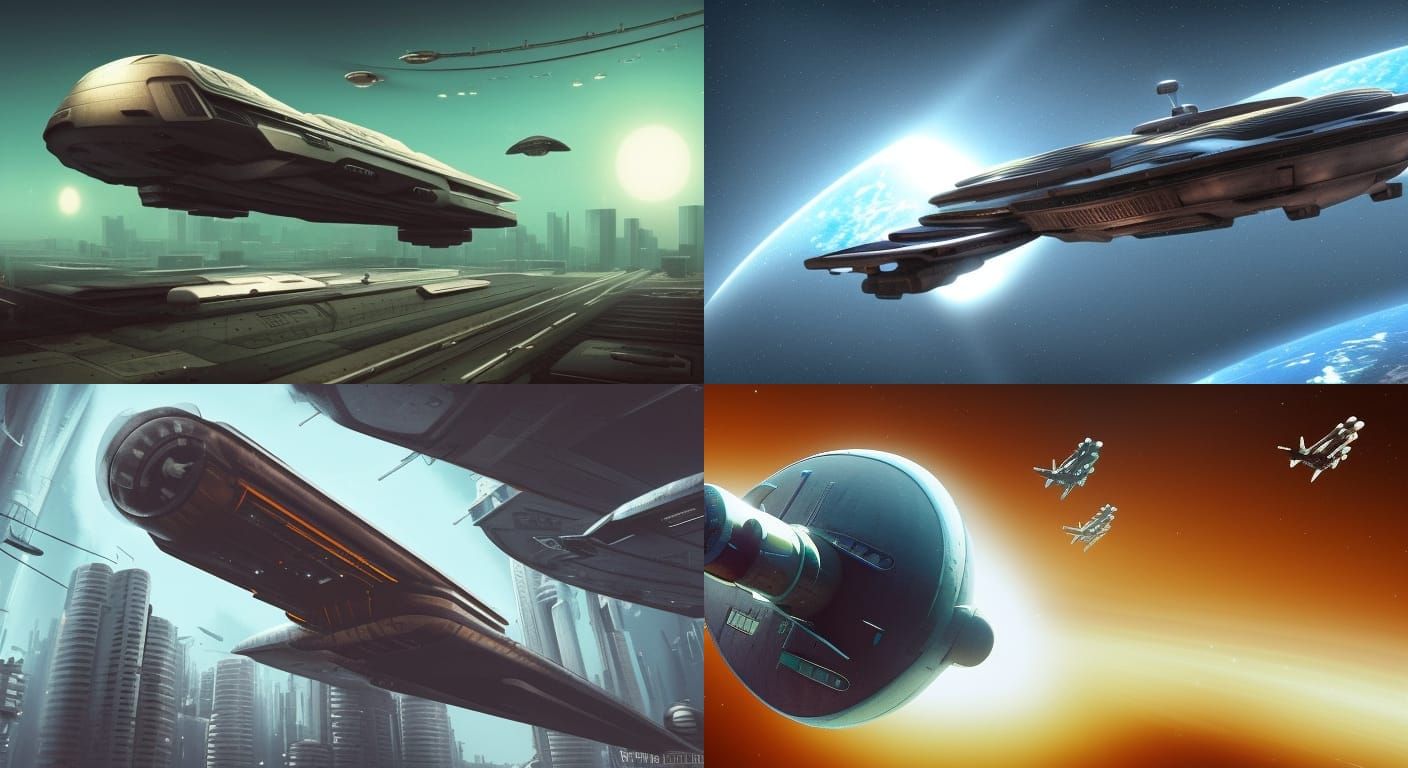The image is split into four distinct sections, each occupying a quarter of the total frame. 

In the upper left section, there's a futuristic flying train, torpedo-shaped with a rounded front, hovering over a road. The background features a sprawling cityscape under a sky with two celestial bodies – one resembling the sun and another akin to the moon. Accompanying the train, several delta wing aircraft soar through the sky, and the area is bathed in a greenish light, suggesting an advanced, high-tech environment.

The upper right section showcases a sleek, flat spacecraft against a gray and white backdrop, seemingly in space. The craft has a disc-like shape with a central tower and a protruding front section, constructed from silvery metal, and the sky in this frame is blue, contrasting with the monochrome space setting.

In the lower left section, another futuristic vessel is depicted, this time with a noticeable long tail ending in a point. The background again features a high-tech city with many tall, round office buildings, giving it a sense of being set in a distant future, potentially around the year 2500 or beyond. There’s a slight orange hue present in this frame.

The lower right section features three flying ships in a brownish background. These ships are encircling a disc-shaped object with a central rod, reminiscent of the International Space Station. The scene is vibrant with various shades of orange dominating the frame, implying a different atmospheric setting compared to the others.

Overall, each quadrant portrays a unique futuristic aircraft in settings ranging from urban cityscapes to outer space, highlighting advanced technology with distinctive glowing lights and metallic structures.